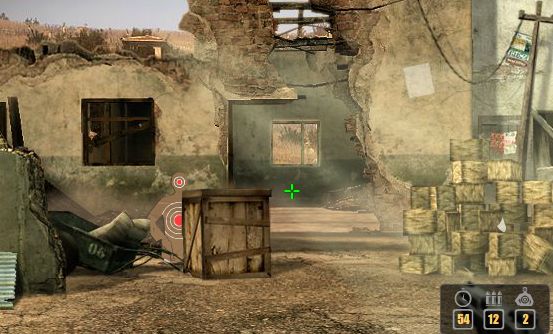The image depicts a screenshot from a shooting video game set in a war-torn, dilapidated environment. Central to the screen is a green crosshair, indicating the player's targeting reticle. The scene features an abandoned, broken house with crates and wooden boxes scattered around. To the left, there is a practice target dummy, beige with red circular holes on its head and stomach, used likely for target practice. In the bottom right corner of the screen, three icons are visible, each with yellow numbers: a stopwatch icon displaying '54', a bullet icon showing '12', and a practice dummy icon with a '2'. The atmosphere is dominated by earthy brown tones, with splashes of green, red, black, blue, and a bit of white. Additionally, there are electrical poles leaning sideways, contributing to the desolate feel of the environment, and a utility cart marked with the number '6'.